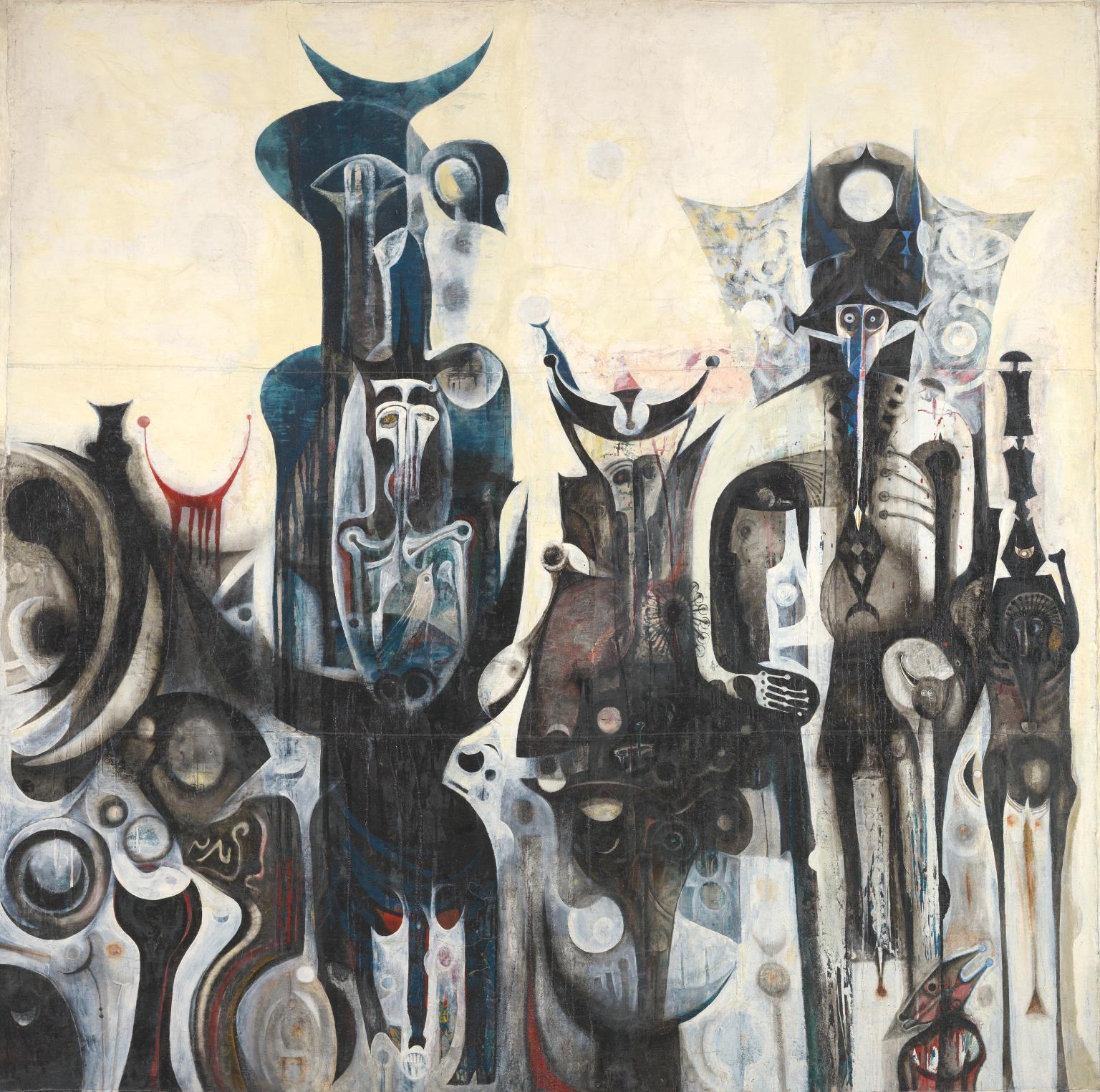The image is an abstract, dark-toned art piece depicting an eerie and intricate collage of humanoid figures mixed with various morphed shapes and symbols. The figures have skeletal and monster-esque features, with droopy eyes and heads that seem to blend into one another, creating an almost indistinguishable mix of forms. Some figures appear to be adorned with masks and shadowy, elaborate clothing. The overall color palette is dominated by black and white, interspersed with occasional dark blue and white highlights. Notably, there is a prominent red element on the side—an ominous half-circle, dripping like blood, which carries a sinister, smiley face appearance. The figures and shapes appear to emerge from and meld into each other, contributing to a chaotic yet cohesive composition, evoking a sense of unsettling mystery and darkness.